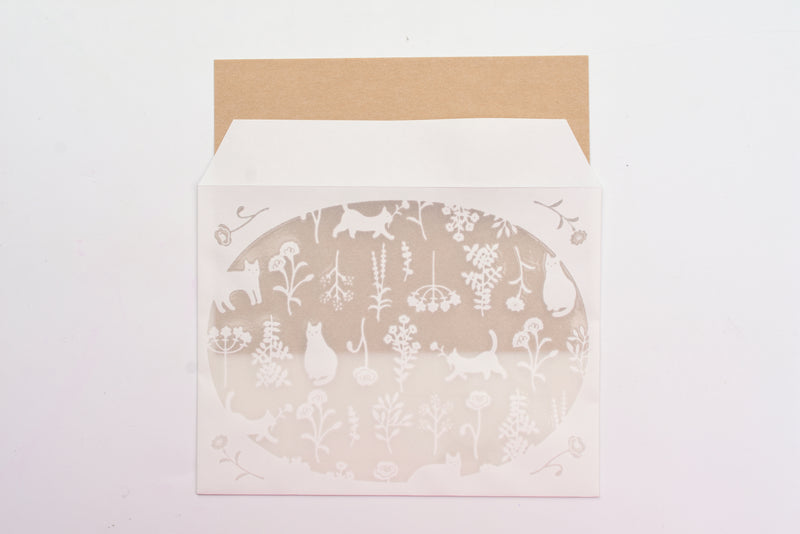This image depicts a delicate, artistic scene centered on a white envelope with an oval cutout in its front. The background of the image features a frosted glass effect, creating a subtle, cloudy layer across the bottom. Through the oval cutout in the envelope, a brown piece of paper is partially visible, enhancing the contrast. The envelope is adorned with intricate white silhouettes of cats in various poses—sitting, standing, walking, and lying down—as well as a mix of flowering and non-flowering plants. These silhouettes give the envelope a detailed and whimsical appearance of paper cutout art. Each corner of the envelope features a standalone rose design in the same sheer material, contributing to the overall pastel pink tone and ethereal quality of the stationary set.